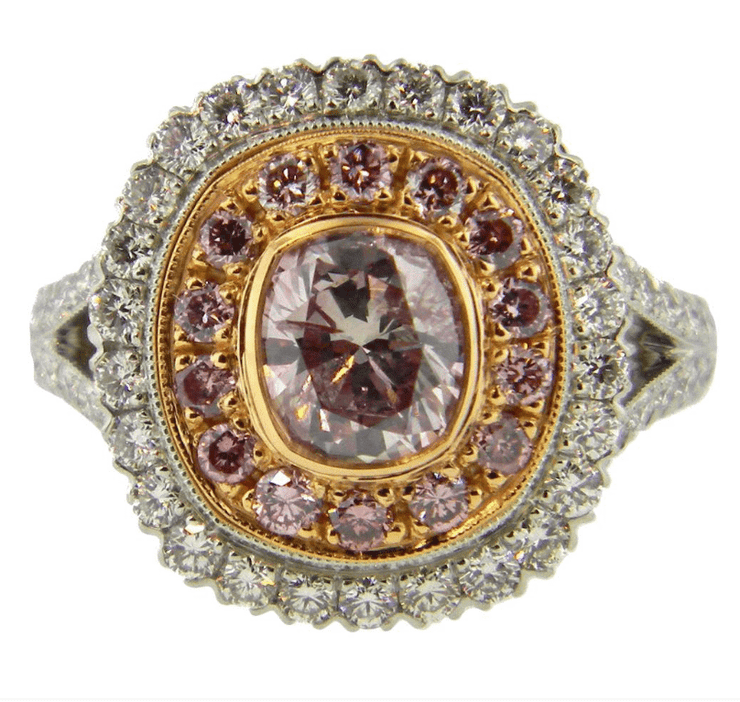This image showcases an opulent and intricately designed ring. The focal point is a very large diamond at the center, which appears to be white with a potential hint of pink or red. Surrounding this central diamond is a circular pattern of small, dark red gemstones—likely rubies—set in a gold background, each secured by four gold brackets.

The face of the ring features a double-layered design: a gold circular section embedded with the red gemstones, encompassed by a broader silver band adorned with white diamonds. The diamonds continue around the circumference of the ring, forming a dazzling, uninterrupted line.

Notably, the face of the ring includes two prominent V-shaped cutouts on each side, adding a unique structural element. The band itself is predominantly white gold, with the center of the ring accented by a black strip flanked by parallel rows of closely set diamonds, enhancing the ring’s luxurious and eye-catching appearance.